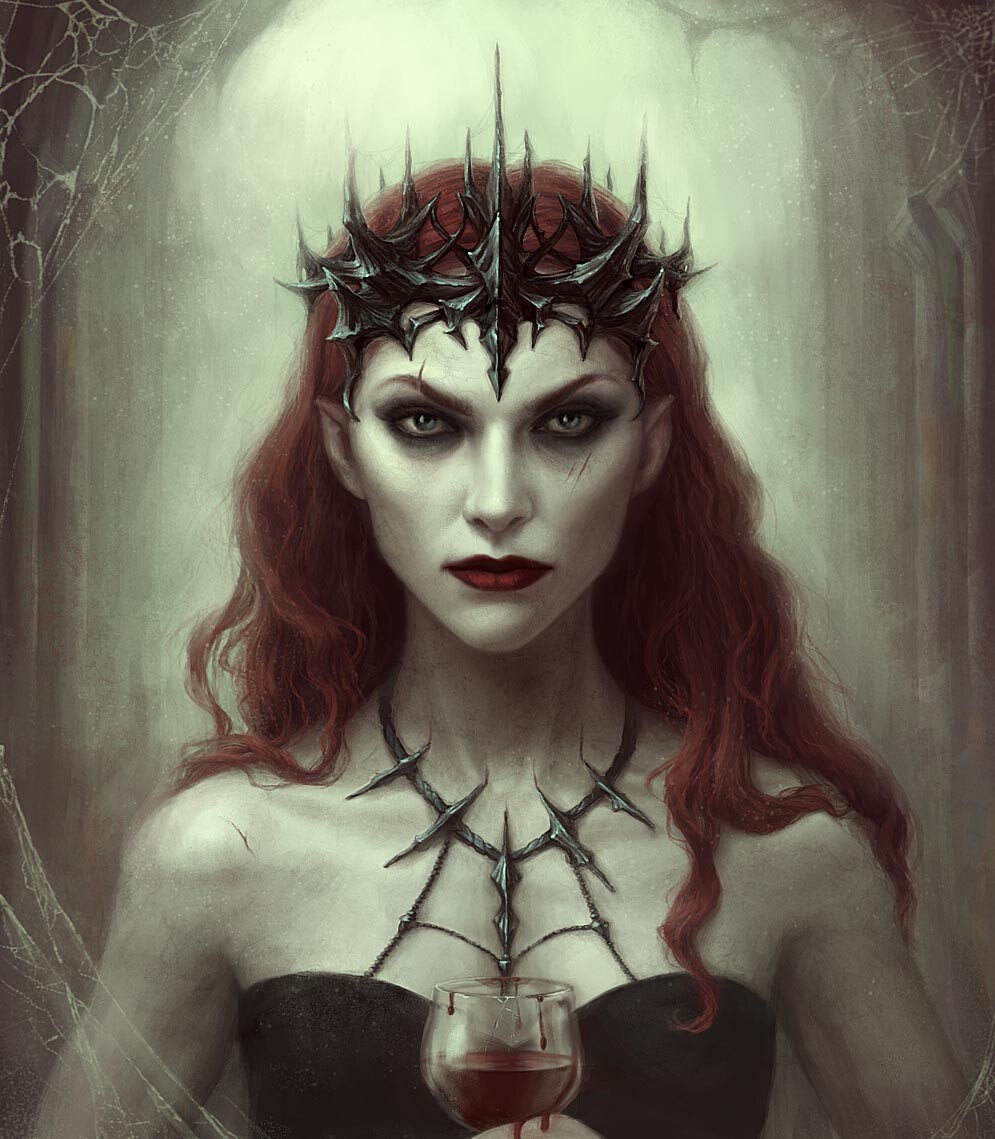This detailed art piece features a striking woman with red hair, possibly a vampire, rendered in either hand-painted or digital medium. Dominating the image, she sports vibrant red lipstick and piercing blue eyes accentuated by dark eyeshadow. Atop her head is a menacing, geometric black crown, and around her neck, she wears a sharp, metallic black necklace. Her attire includes a strapless black dress, revealing her pale white skin and slender figure. In the bottom center of the image, she holds a glass with a thick red liquid, possibly wine or blood, which drips ominously from the rim. The background portrays a dimly lit corridor or archway with spider webs intricately woven into all four corners, using a color palette of mostly red, mint green, and varying shades of black and white to create a dark, eerie atmosphere.